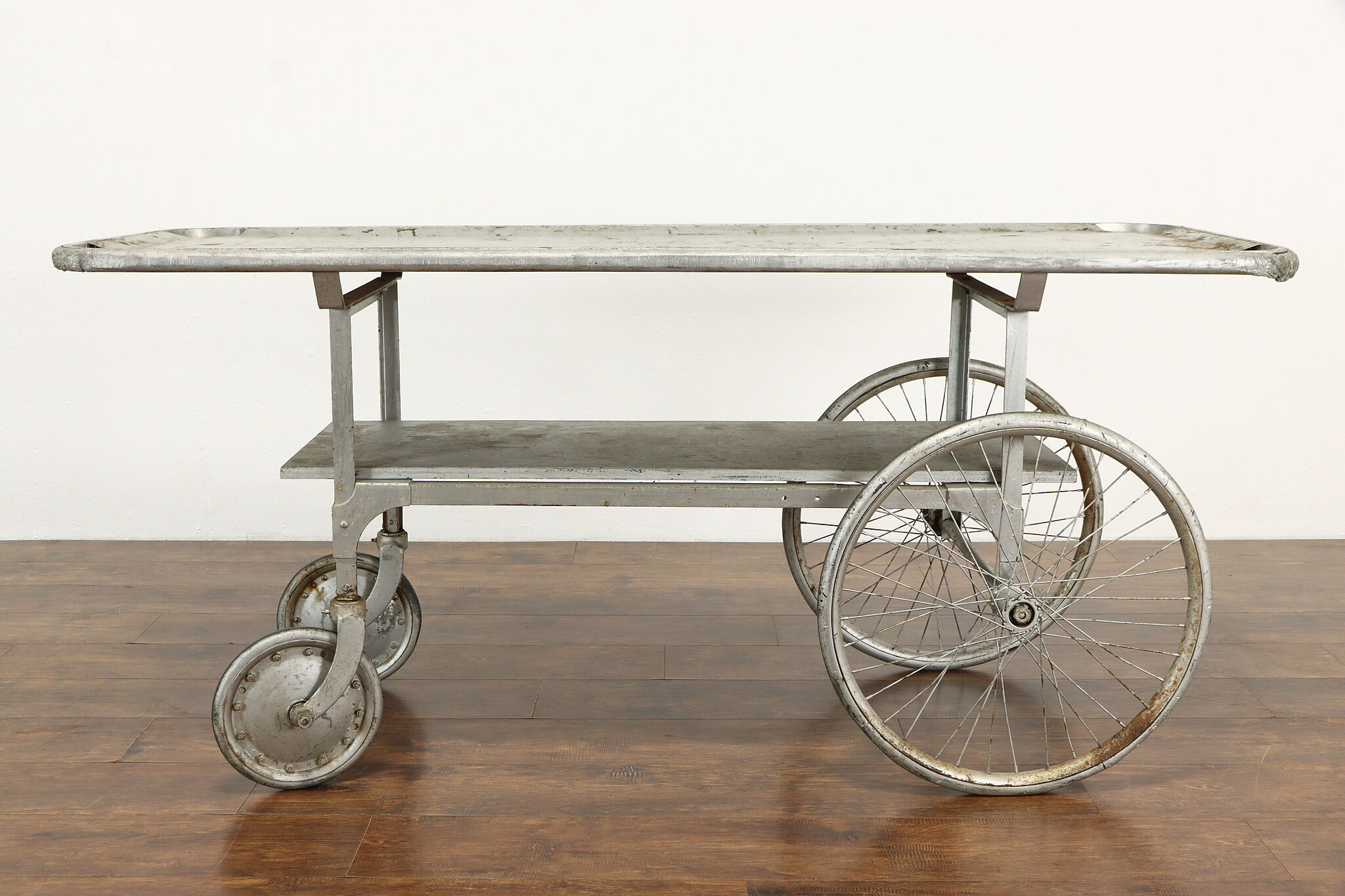This photograph features a vintage stainless steel cart, reminiscent of those used in hospitals or mortuaries. The cart is distinctly old, evidenced by its design and the dirt and rust adorning its surface. It has a sturdy frame consisting of two trays: a middle tray and a flat top tray with a raised rim, likely intended to contain any fluids. The cart is equipped with two sets of wheels—larger, bicycle-like spoked wheels at the rear and smaller, fully solid metal wheels with circular bolts at the front. The entire structure, including the wheels, is made of metal. The backdrop is a stark white wall, and the cart sits on dark, shiny, hardwood floors with its shadow clearly visible.